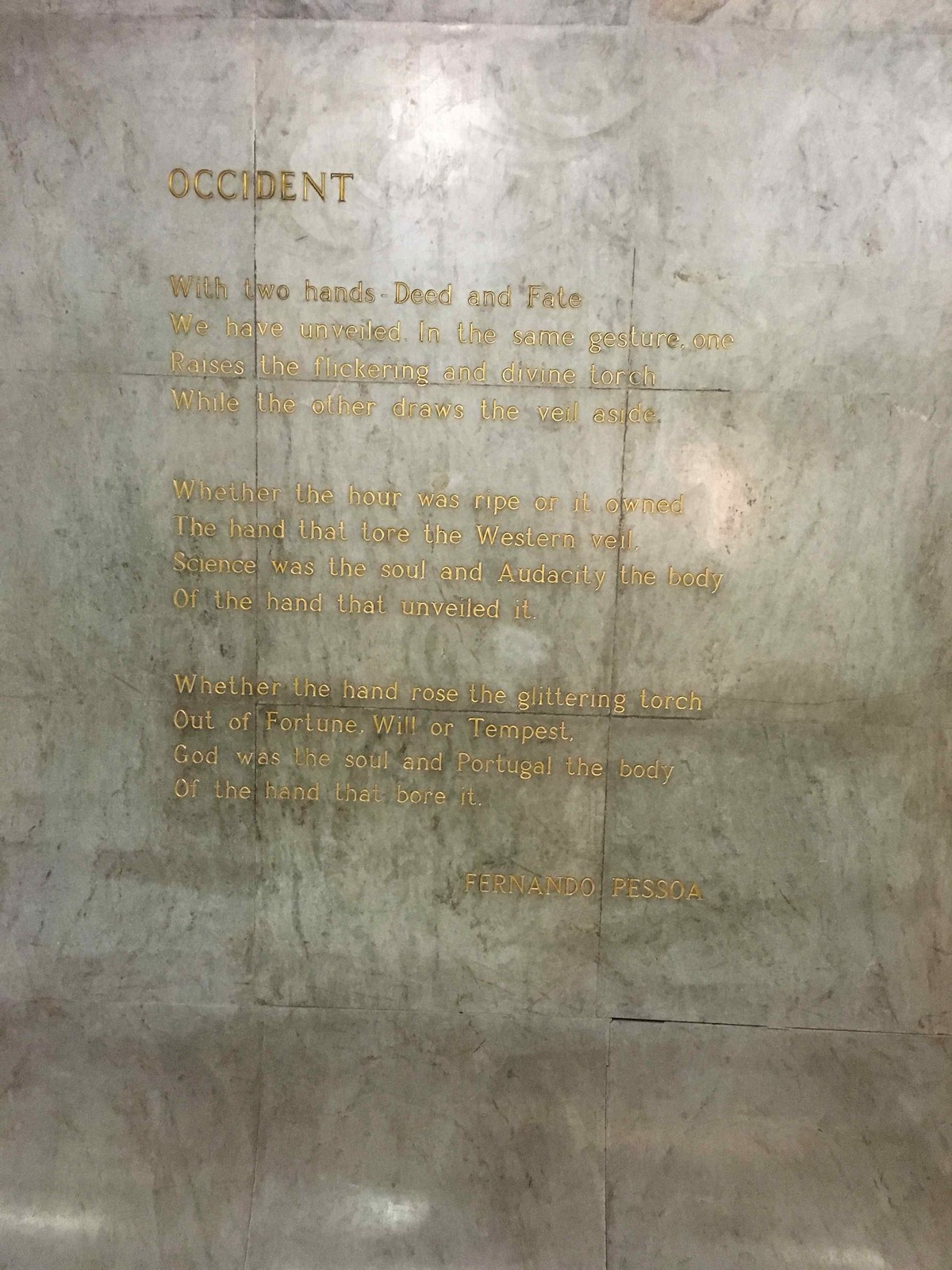This image showcases a tall, rectangular marble floor in pearl and gray hues, consisting of large square tiles arranged in a grid-like pattern of three columns and four rows. The marble surface, adorned with intricate gray veins, exudes a subtle shine. Featured prominently at the top in golden engraved, all-capital letters is the word "OCCIDENT." Below, in a more refined gold font, is a poem by Fernando Pessoa. The verse, written in three stanzas, reads: "With two hands, deed and fate, we have unveiled in the same gesture one raises the flickering and divine torch while the other draws the vast veil aside whether the hour was ripe or it owns the hand that tore the western veil science was the soul and audacity the body of the hand that unveiled it whether the hand rose the glittering torch out of fortune will or tempest god was the soul and Portugal the body of the hand that bore it." The overall appearance conveys a blend of artistic elegance and literary depth, enhanced by the polished marble and gleaming gold script.